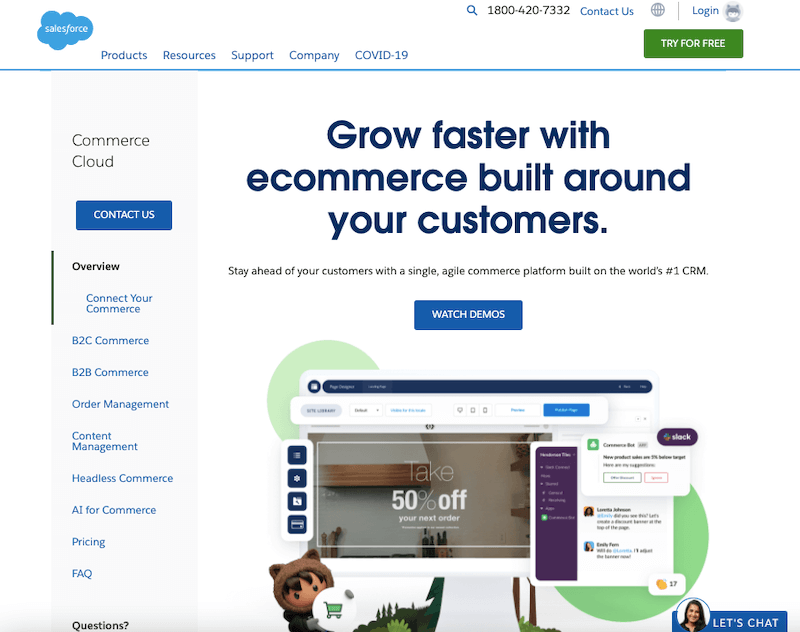This screenshot showcases the homepage of a company's Salesforce Commerce Cloud platform. The top navigation bar includes sections for "Products," "Resources," "Support," "Company," "COVID-19," a button to "Try for Free," an option to "Log In," and a "Contact Us" link, alongside a customer service phone number, 1-800-420-7332.

On the left-hand side, a vertical menu provides an overview of the webpage and includes links for "Commerce Cloud," "Contact Us," "Overview," "Connect Your Commerce," "B2C Commerce," "B2B Commerce," "Order Management," "Content Management," "Headless Commerce," "AI for Commerce," "Pricing," and "FAQ."

Central to the page, promotional text encourages users to "Grow Faster with E-commerce," "Build Around Your Customers," and "Stay Ahead of Your Customers." Beneath this, there are demo videos showcasing various features and functionalities of the platform.

Additionally, in the bottom-right corner, there is a chat box labeled "Let's Chat," designed in a vibrant color scheme of blues and greens. This area features a cartoon-styled avatar, enhancing the user-friendly and approachable aesthetic of the website.